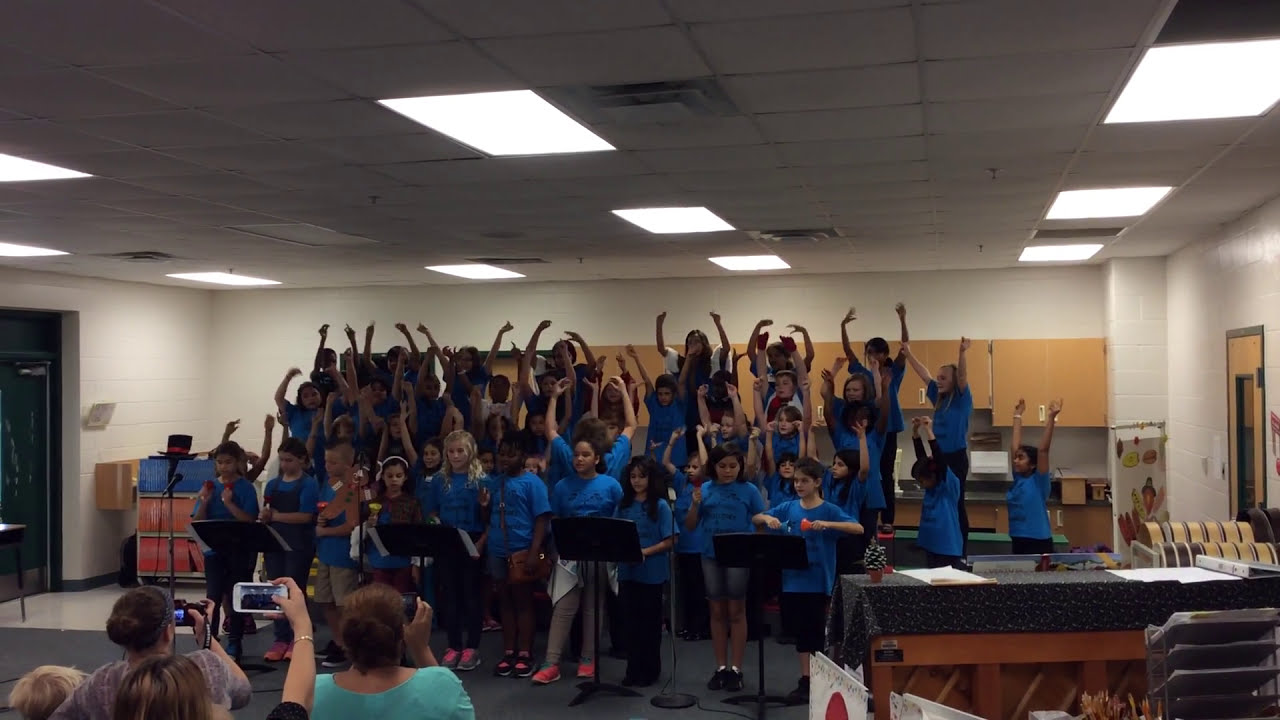This photograph captures a vibrant choir classroom filled with young girls, approximately 7 to 9 years old, all dressed in matching ocean blue short-sleeved t-shirts. The girls exhibit a variety of bottoms, with some wearing shorts, jeans, or sweatpants. Positioned in neat rows, with some on elevated platforms, most of the children have their hands raised as part of their spirited performance. The classroom, with its white cinderblock walls and recessed ceiling lights, includes musical instruments like a piano and guitars, and the scene is animated by the presence of parents in the foreground, eagerly capturing the moment with cameras and video recorders. Front-row sheet music stands and a colorful red and blue orange cart add to the organized yet lively atmosphere of this large, bustling classroom.